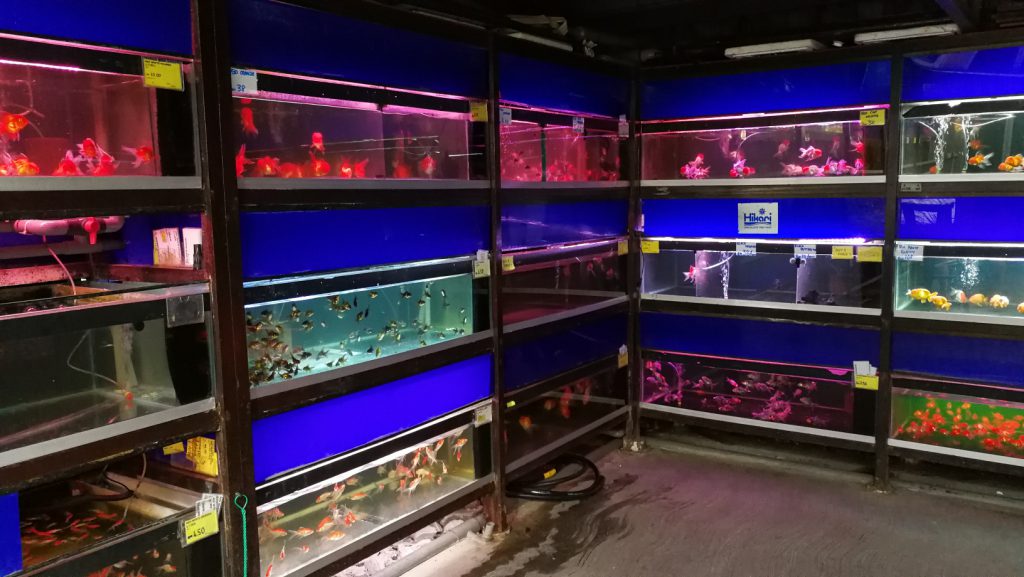Captured in an indoor pet store, this detailed image showcases a typical bustling scene centered around a series of built-in aquariums. The concrete floor, wet from a leaked black water hose coiled haphazardly, reflects a sense of disarray near the aquariums displayed centrally. Aquariums are embedded into the wall, interspersed with striking blue gaps, and adorned with vibrant yellow price tags. The top rows of aquariums are illuminated with purple lights, casting a unique purple hue across the tanks. Notably, the aquarium on the right features a lively spectrum of aquatic life, with orange fish swimming at the bottom, yellow fish in the mid-section, and a lighter shade of orange fish near the top. On the left side of the image, green cables hang loosely alongside a green fish net, hinting at the tools of the trade in this aquatic haven.